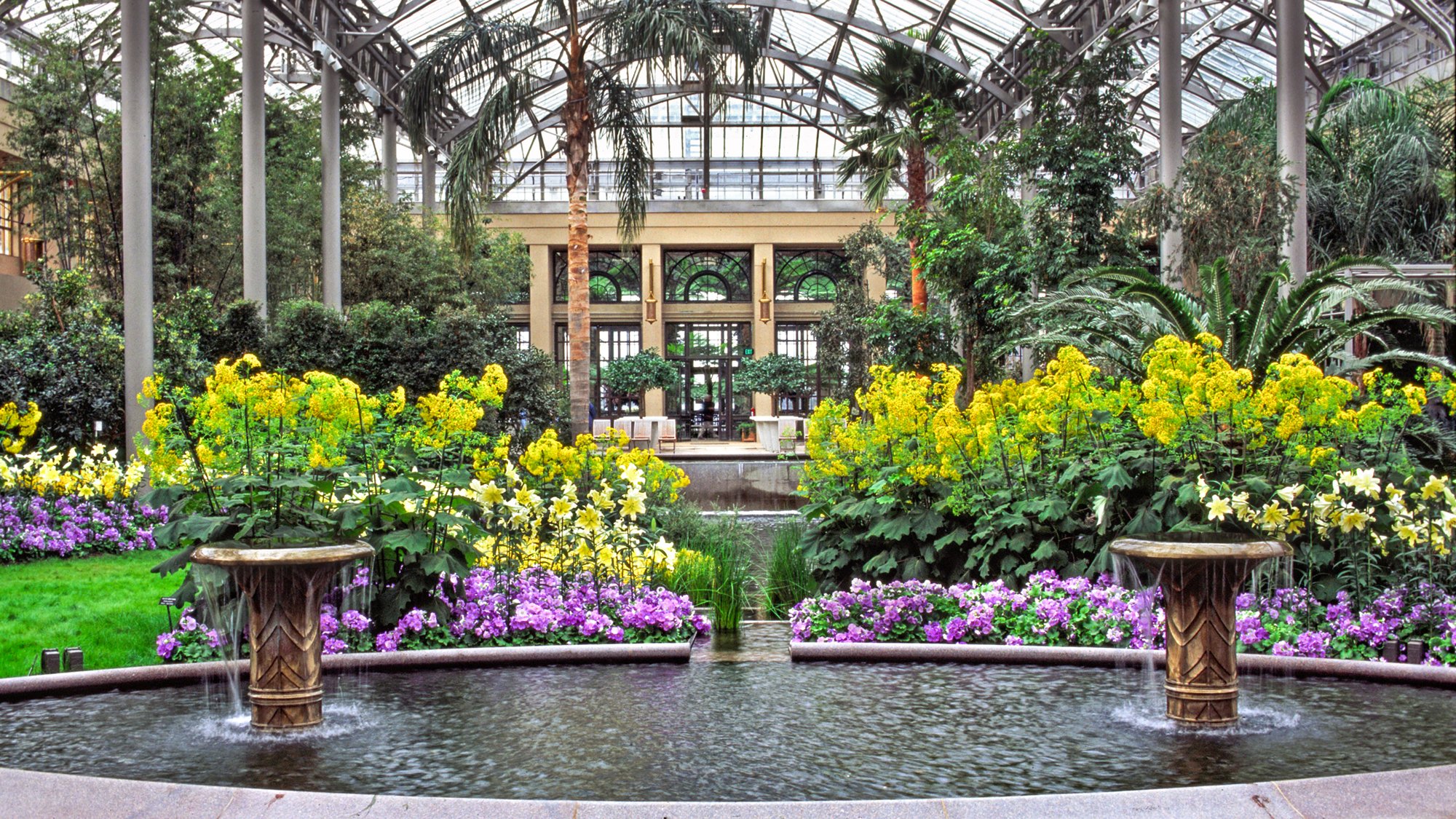This photograph captures an expansive indoor garden within a large greenhouse, characterized by its fully glass ceiling that allows natural light to illuminate the vibrant greenery. The layout features symmetrical elements, including two prominent water fountains facing each other, which serve as focal points in the foreground. These fountains appear to be circular or oval in shape, with light brown pedestals extending from the water and supporting plants from which water gently drips back into the pool below. Surrounding the fountains are various colorful plants, including lush pink flowers in the immediate vicinity, and further back, a mix of yellow blooms, blue, and white flowers, creating a vibrant palette. A grassy area interspersed with more pink flowers extends towards the background, where larger green trees and bushes add depth to the scene. Supporting pillars hold up the glass ceiling, giving the space an airy and open feel. In the foreground, there is a small stage area that suggests the space could be used for events such as weddings. The glass-encased arches in the distance offer a glimpse of the exterior, blending the indoor and outdoor environments seamlessly. The overall tranquil atmosphere is enhanced by an overcast sky, indicated by the absence of direct sunlight streaming through the glass.